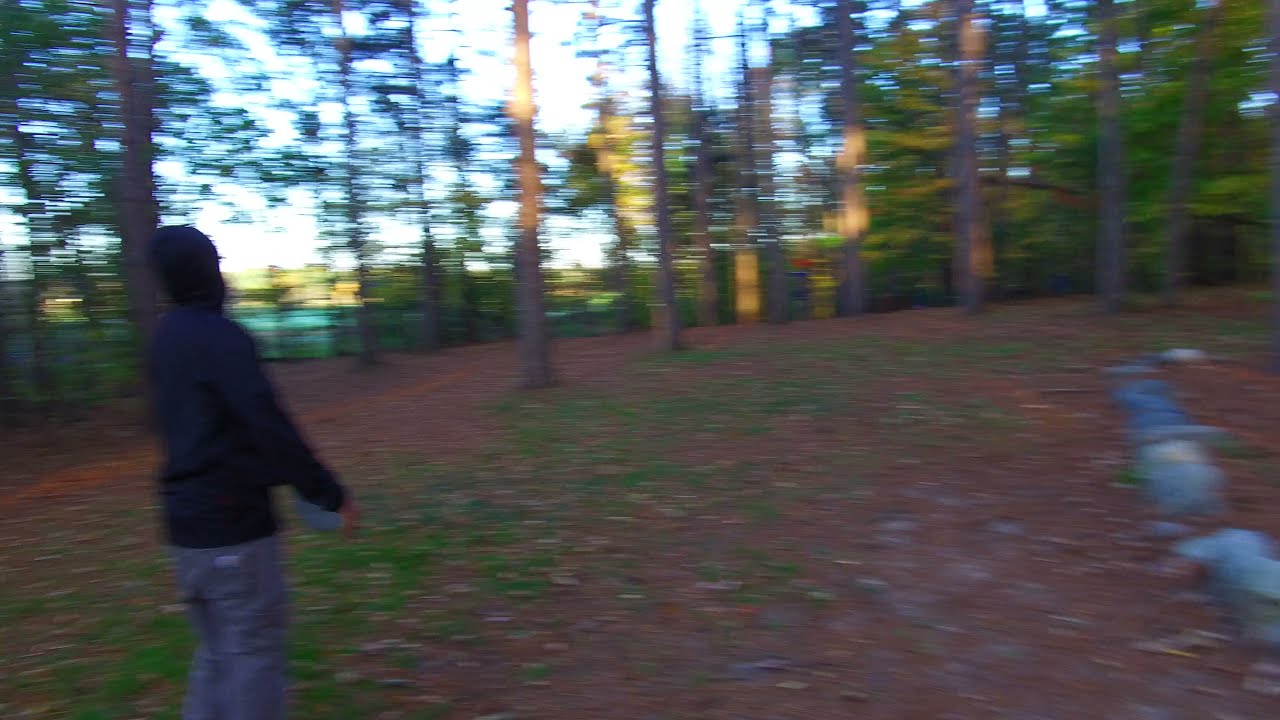The image depicts a blurry, sunny scene, likely caused by the photographer’s quick movement to the left while capturing the picture. It shows a man standing on the left side of a relatively barren, forested area. He is seen from the back, clad in a black hoodie and jeans. The ground beneath him is a mix of patchy grass, clay-like dirt, and scattered leaves. In the backdrop, there are numerous tall, healthy-looking trees, behind which a clear blue lake can be faintly discerned on the far left. Despite the blur, the sky appears blue, indicating it's a bright, clear day. The entire setting, though wooded, is not densely packed with trees, creating a patchy, open space where the man stands, seemingly observing the distant scenery.